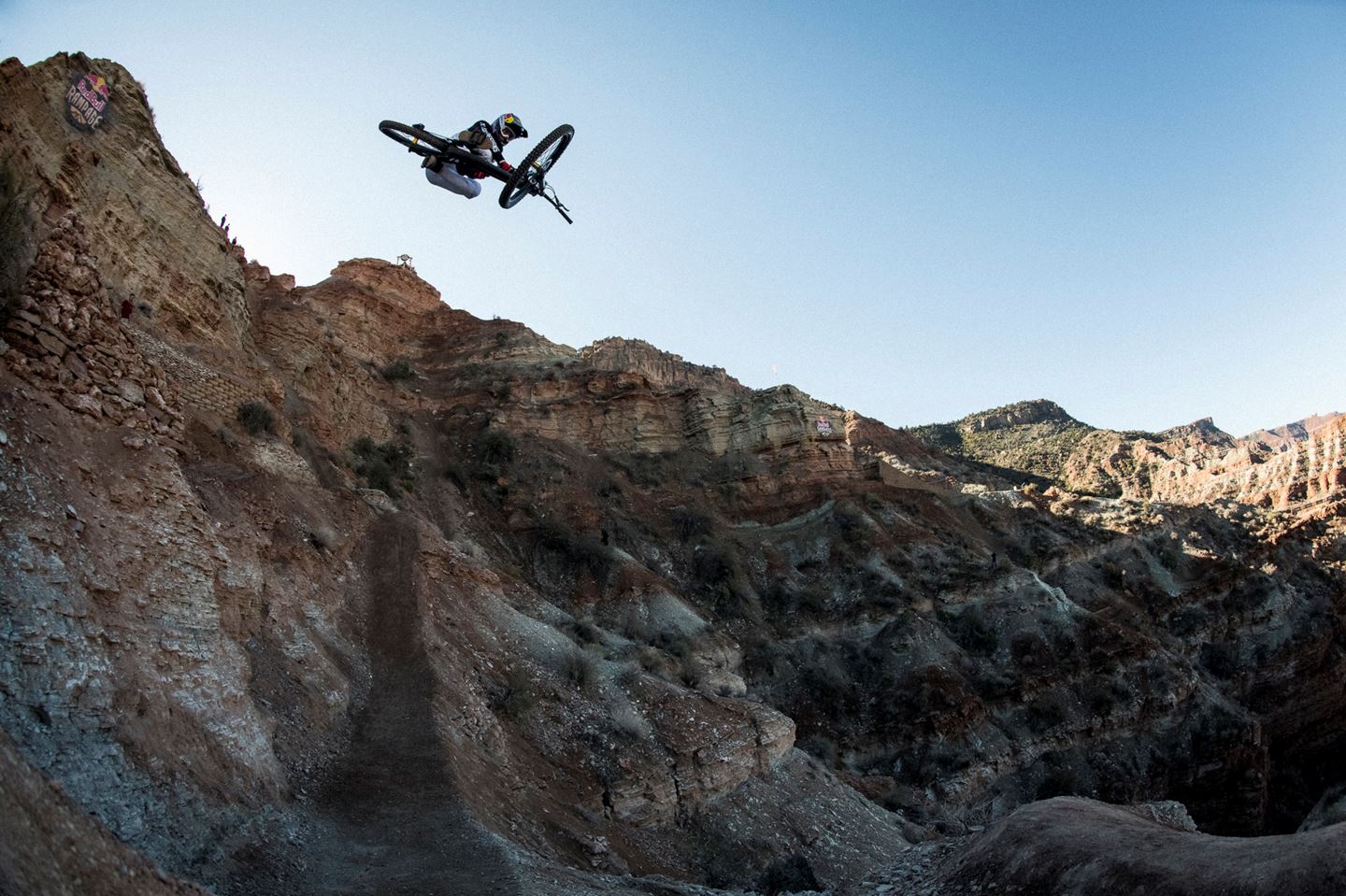The image captures a dramatic scene of a professional biker executing a daring stunt off the edge of a steep, rocky mountain cliff. The landscape is dominated by large brown, white, and gray rocks with sporadic bushes and dirt trails weaving through the arid terrain. In the center of the picture, slightly off to the left, a dirt path ascends and abruptly ends at the precipice from which the biker has launched. The biker, clad in a black long-sleeved shirt, gray pants, and a black, yellow, and white helmet, is airborne with his black bike tilted mid-maneuver. Far in the background, the bright blue sky is dotted with a few clouds, enhancing the sense of height and openness. There is also a hint of some bricks and man-made structures atop the mountain, adding to the rugged and adventurous atmosphere. A drone or some other device might be capturing this breathtaking moment from above, emphasizing the professional and high-intensity nature of the stunt.